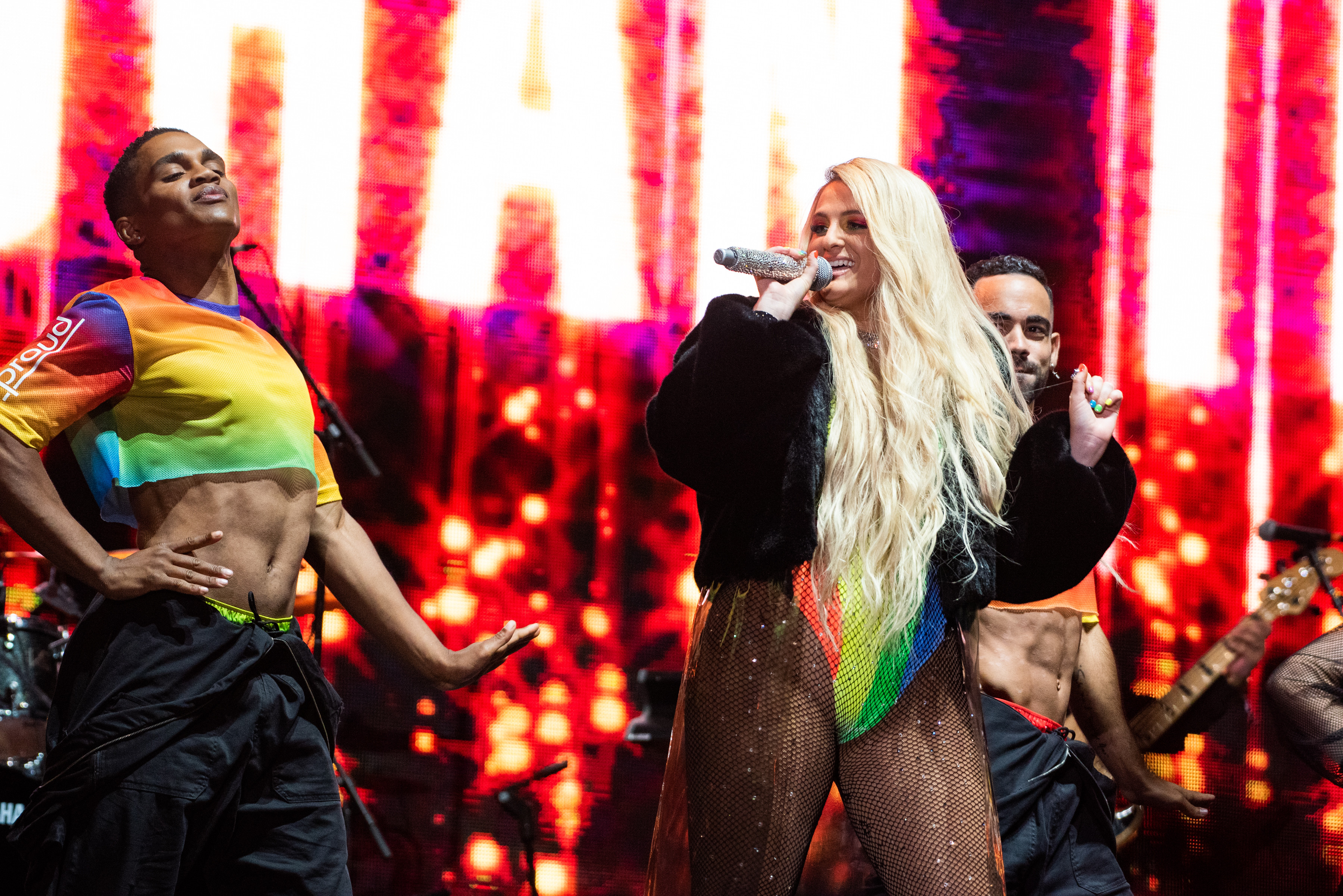This vibrant color photograph captures a lively stage performance featuring three key performers. On the left, a man strikes a dance pose, his right hand on his hip while his head is tossed back, showcasing his black hair. He wears dark baggy pants and a rainbow-colored cut-off T-shirt with the word "Proud" in white text on the sleeve. To his right, a woman with very long, bushy blonde hair holds a sparkly microphone to her mouth. She is dressed in a black jacket over a rainbow-colored swimsuit, paired with fishnet stockings and a sheer skirt. Behind her, slightly to the right, stands another man mirroring the first man's outfit of a rainbow top and dark pants, looking at the woman. In the background, several musicians are partially visible, including guitar players and a drum set located on the left side of the stage. A bold, illuminated sign with large, unreadable white letters and blinking red lights on a black background creates an electrifying atmosphere behind them.